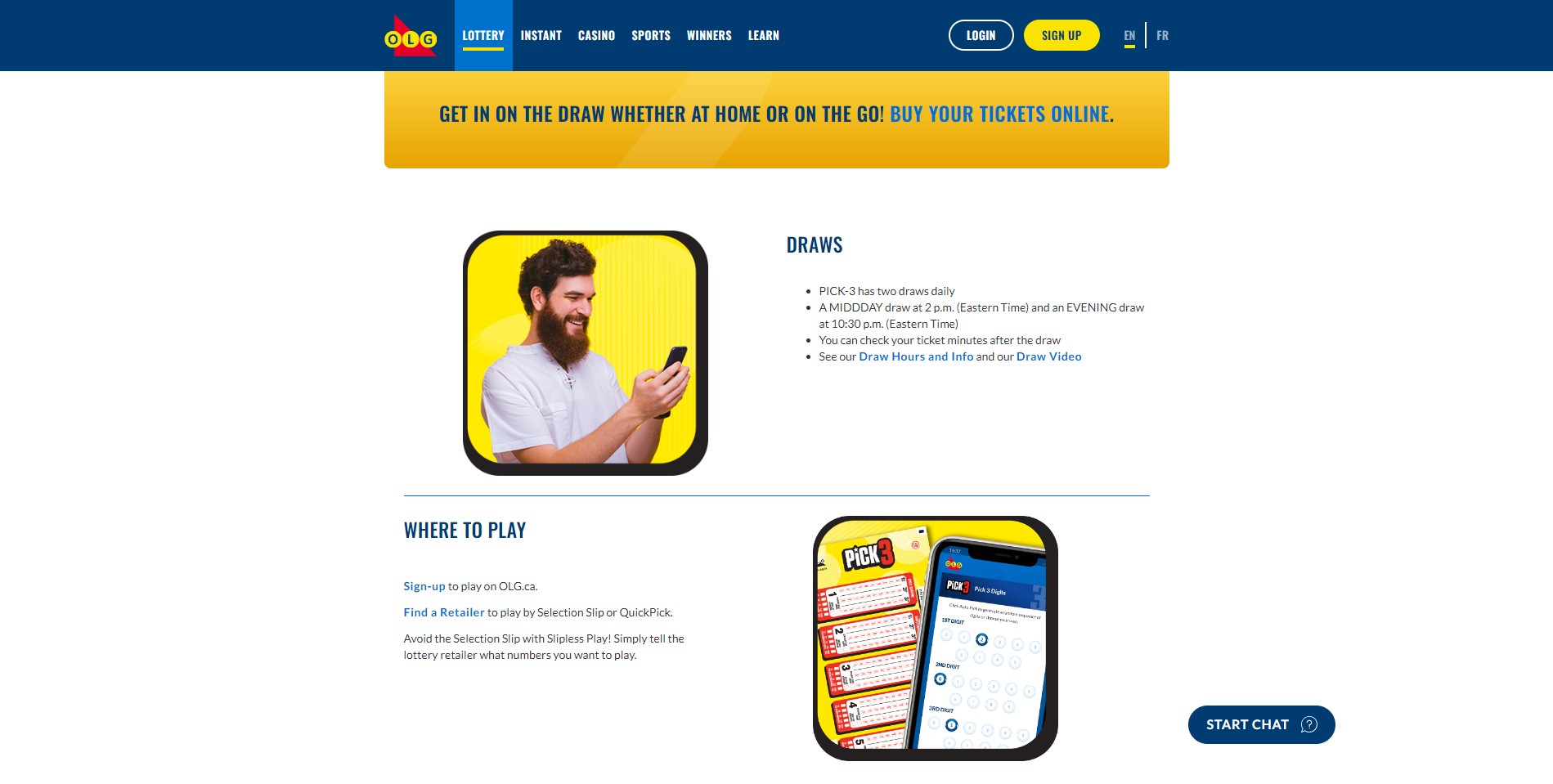**Caption:**

This detailed screenshot, taken from the OLG Lottery website, showcases various sections and features aimed at lottery enthusiasts. In the upper left-hand corner, the navigation menu provides quick access to different categories such as "Instant Casino," "Sports," "Winners," "Learn," "Login," and "Sign Up." 

Below the menu, a prominent banner encourages users to participate in the draws, either from the comfort of their homes or on the go, by purchasing tickets online. Specifically, the "Pick Three" lottery offers two daily draws: a midday draw at 2:00 PM Eastern Time and an evening draw at 10:30 PM Eastern Time. Users can check their tickets shortly after the draw and are provided with details on draw hours, information, and videos.

Additionally, the screenshot informs users about various ways to play, including signing up on OLG.ca, finding a retailer, using a selection slip or opting for a quick pick. It highlights the convenience of "Slipless Pay," where players can simply tell the lottery retailer their chosen numbers.

The entire image is framed within a rectangular shape, making it visually clear and easy to read.